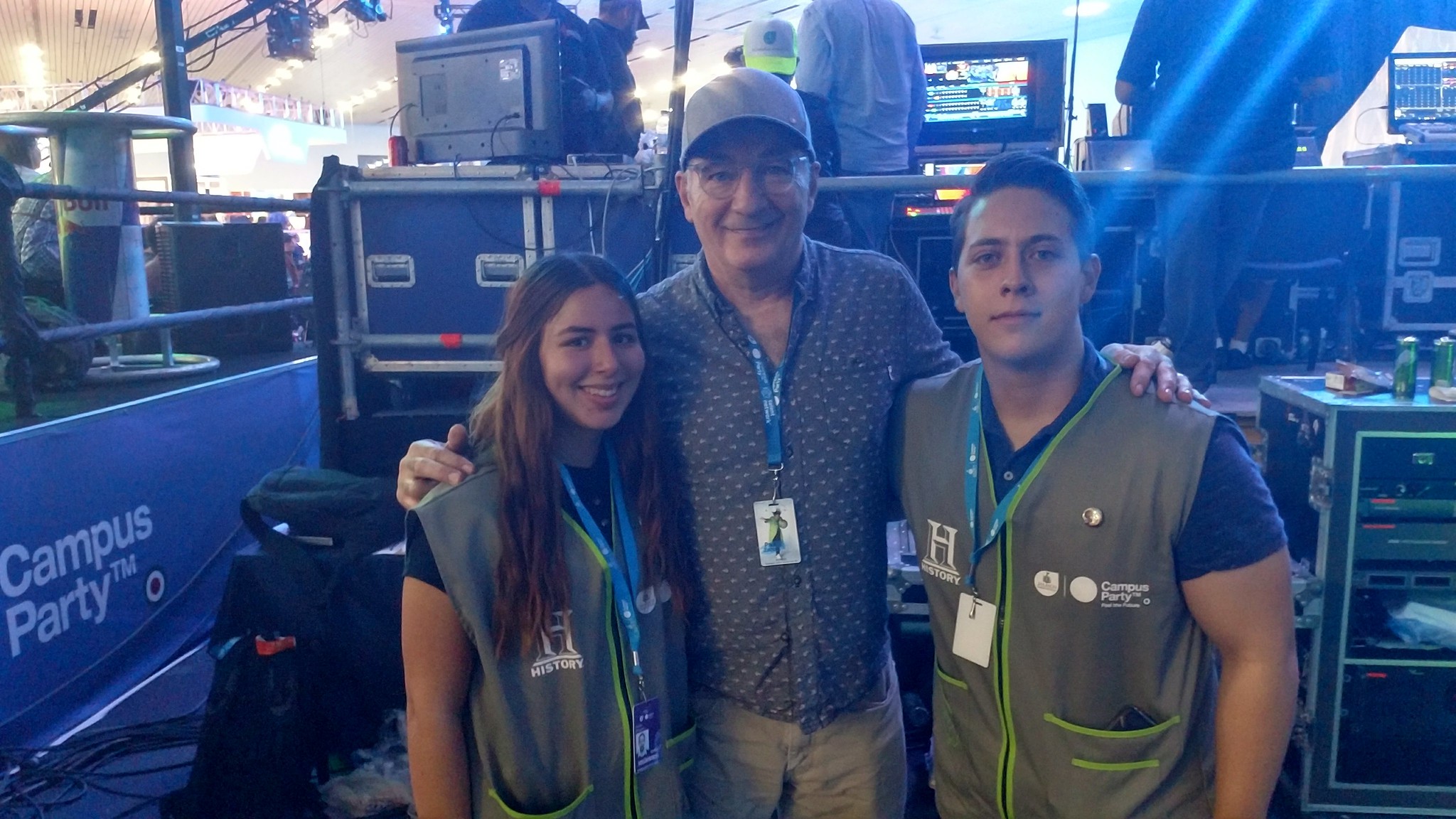The photograph captures a lively backstage scene at a large, well-lit event, possibly in a vast auditorium judging by the tall ceiling visible in the background. The setting features a stage setup brimming with DJ equipment, computer screens, cords, and lighting gear, seen in the distance on an elevated platform. In the foreground, three people pose for the camera: a middle-aged man in the center with gray attire, including a hat, shirt, and light pants, and an identification badge around his neck, displaying a warm smile with his hands resting on the shoulders of a young woman and a young man beside him. The young woman, with long brown hair, is dressed in a gray vest over a black t-shirt, while the young man, sporting short dark hair, wears a similar vest and dark t-shirt. Both also have name tags around their necks. All three individuals are smiling, conveying a sense of camaraderie and enthusiasm. Additionally, the left side of the image has text that reads "Campus Party," indicating the event's name.